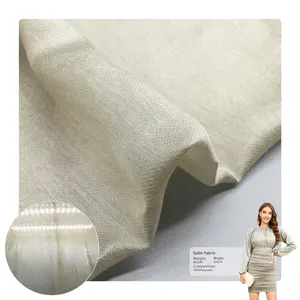The image showcases a piece of off-white fabric, possibly a dress, laid flat on a light grey surface, with subtle folds adding depth. The texture is highlighted, showing slight variations in shading and fine details, including a small circular zoom-in that emphasizes these textures. In the lower right corner, a woman, seemingly the focal point, stands wearing a long-sleeved dress that matches the fabric's color. She has slightly reddish or brown hair, cascading over her shoulders, and holds a white sheet of paper. One hand rests on her hip, while the other hangs down, giving her a poised and confident stance. There is also a tiny, unreadable tag or writing to the left of her, adding a subtle detail to the overall composition. The woman's presence and the fabric's intricate texture suggest a promotional or fashion-related context.